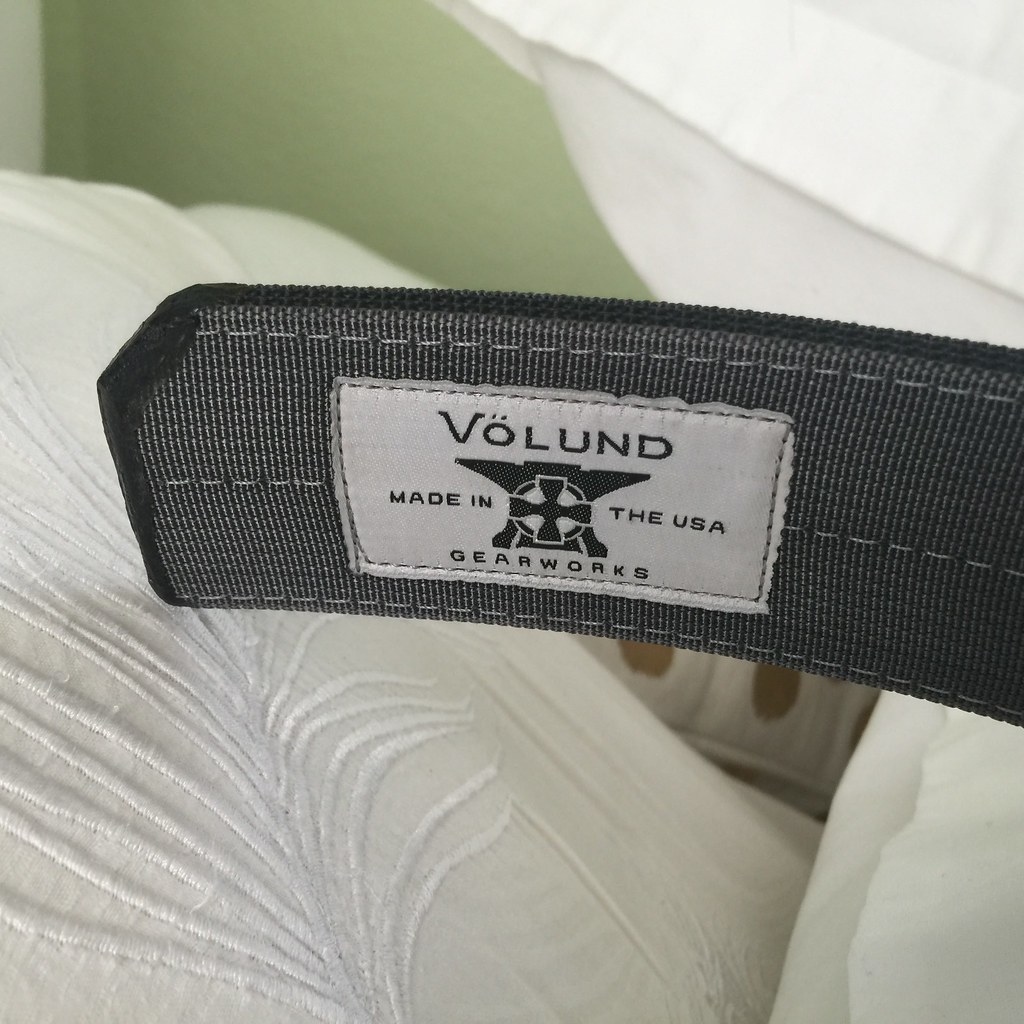This photograph features the inside label of a wide, tactical belt or strap resting on a bed. The belt boasts a distinctive black outline and white stitching along both edges and the middle, set against a gray inner fabric. The label is white or off-white and prominently displays the brand "Volund Gear Works" with an anvil logo that includes a black cross in the middle, accompanied by "Made in the USA." The scene is set against what appears to be a white embroidered pillowcase on a bed, with a green wall and white curtains visible in the background. Additional white fabric with brown circles peeks into the frame from the bottom right.